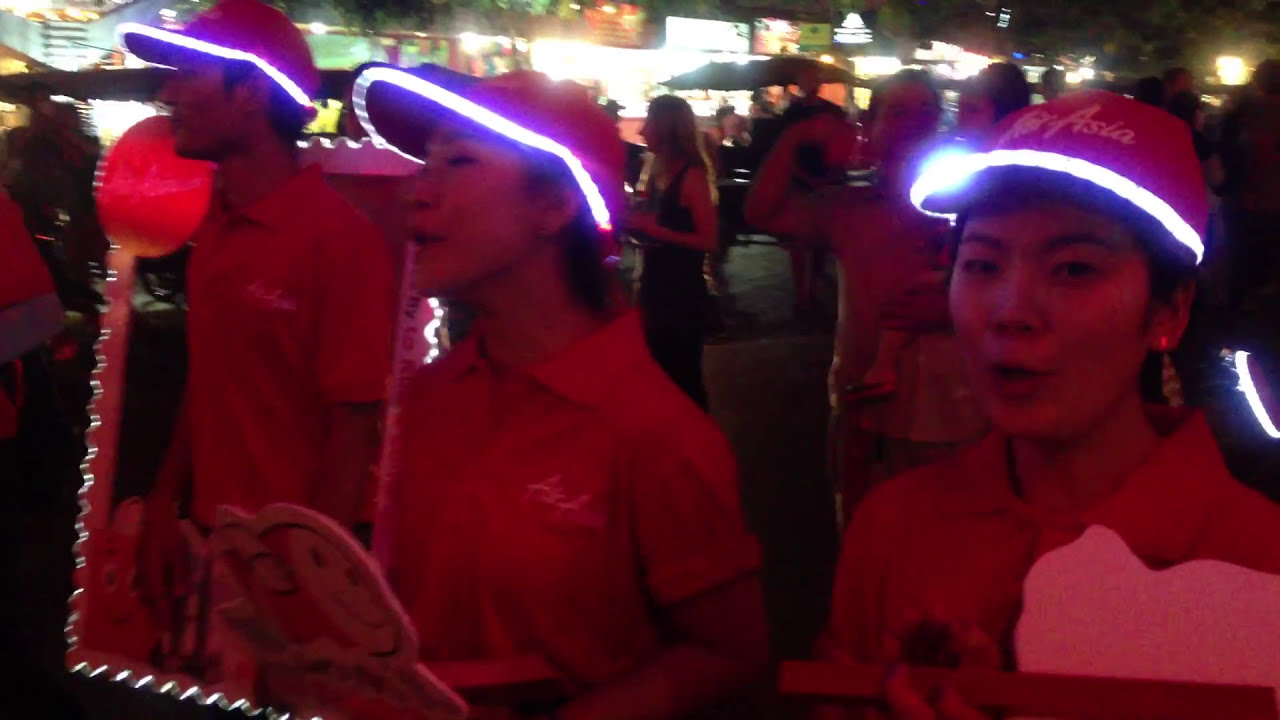The photo captures a side view of three Asian individuals—two women and one man—standing in a line, slightly angled to the left. They are wearing visor hats adorned with glowing white neon stripes around the brims, which creates an illusion of red due to the lighting. Each person is dressed in a pink or red collared polo shirt with illegible white text over the left breast pocket. The hats appear to feature blue brims and some white text, possibly related to Asia. The women seem animated, possibly talking or singing, and hold cut-out cardboard pictures resembling characters like a monkey or bunny. In stark contrast, the man stands still with his hands at his sides.

The setting appears to be an amusement park or carnival, bustling with people and illuminated by bright lights. In the background, there are tables, glowing buildings, facades, and umbrellas, all contributing to a lively and crowded night-time atmosphere. Additionally, the scene features a red ball and a red and white striped pole, although the specific details of these objects are unclear due to the lighting conditions.